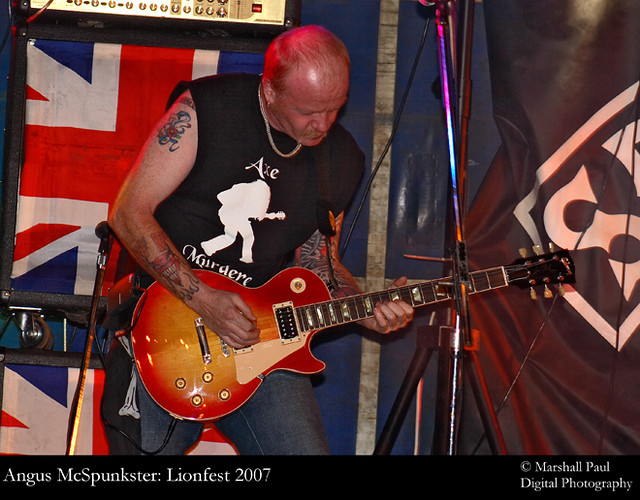This square image captures an older, slightly sunburned white musician deeply engrossed in his performance, bent over as he strums a guitar with a brown base. He is dressed in a black sleeveless shirt, its sleeves seemingly cut off, featuring a white silhouetted guitarist and the words "AXE murderer" emblazoned on it. His mostly bald head shows just a patch of hair on the sides and top. The musician's attire includes blue jeans and tattoos adorning both of his arms, reinforcing his hard rocker persona. Behind him, a British flag (red, white, and blue) is prominently displayed, alongside a partially visible black flag with a white rectangle containing some illegible text due to being cut off by the edge of the image. Around him, various microphone stands and other stage equipment are visible, hinting at a live performance setting. At the very bottom of the image, a black border with white text reads "Angus McSpunkster: Lion Fest 2007," accompanied by a copyright symbol and the words "Marshall Paul digital photography" on the right-hand side.